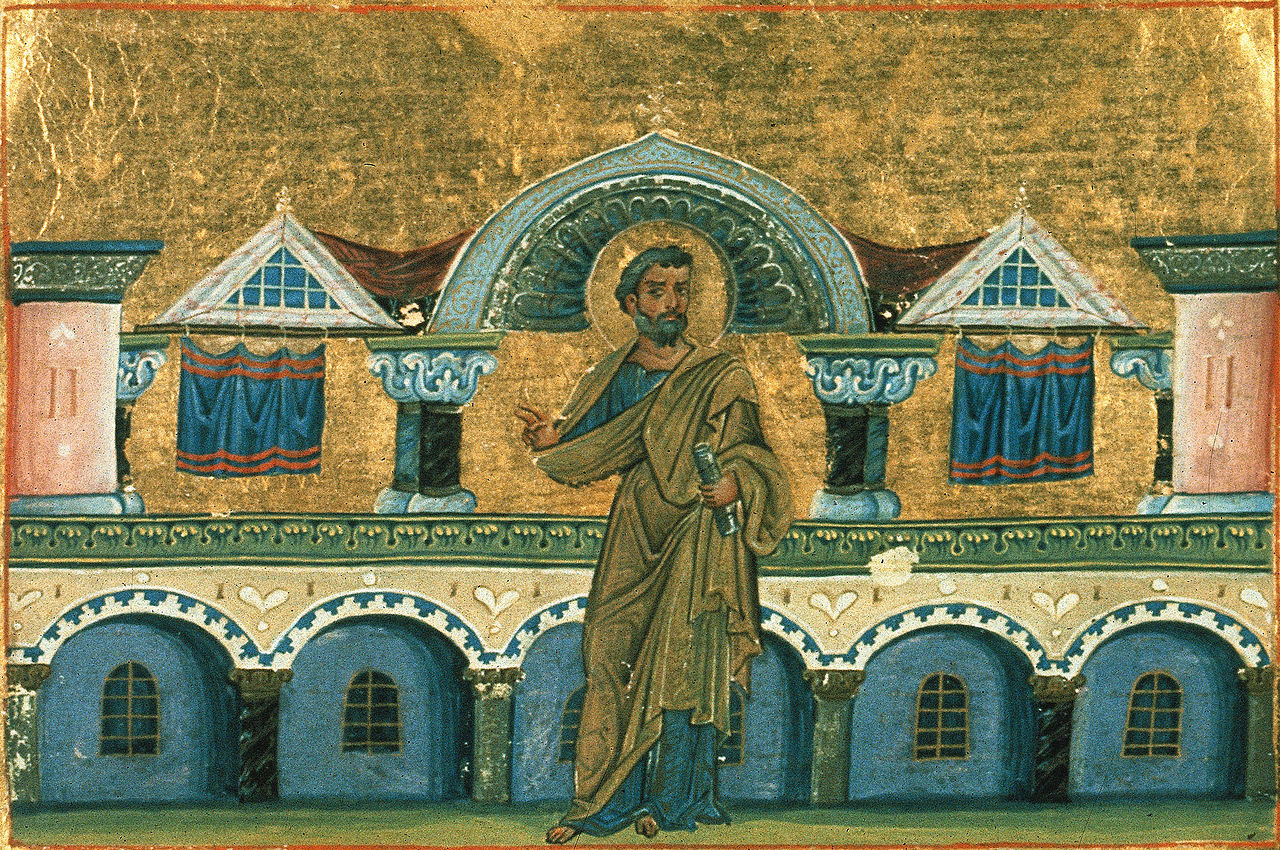The image resembles a detailed painting or intricate drawing, prominently depicting a figure that evokes the likeness of Jesus. He stands in the center, draped in layered robes—a beige outer layer with a blue one underneath—holding an indistinguishable object in his right hand. A halo encircles his head, accentuating his serene expression, framed by dark hair, a beard, and a mustache. His skin is dark, and his gaze is directed towards the left.

Behind him looms an antiquated, Romanesque building, characterized by its two distinct levels. The lower level features a row of blue arched doorways, while the upper level displays beige walls flanked by red columns on either side. The roof is architecturally unique, combining two triangular sections and a central rounded area above the man's head. The ground he stands on is green, likely representing grass.

The sky or background further amplifies the scene's vividness with a yellowish hue, blending into hints of greenish gray and orange above the ancient structure. Overall, the composition blends classical architecture with a serene, almost sacred atmosphere.